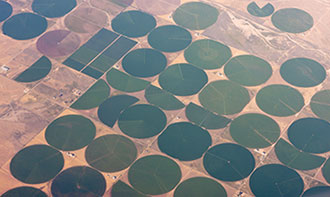This overhead image captures a tiled floor (or possibly an abstract, computer-generated depiction) with a mosaic of various designs. The photograph reveals a blend of tan and marble-like tiles interspersed with prominently featured large, dark-colored circles. These circular patterns are irregular, with many appearing as half or broken circles, giving an unfinished and somewhat chaotic appearance. Towards the bottom center and extending to the left and right edges, several mismatched tiles break the continuity, including a distinct square tile that disrupts the otherwise circular theme. Additionally, there are noticeable gaps in the tiling, particularly on the top left and top right, revealing unadorned sections of floor, further contributing to the overall disordered aesthetic. The image also suggests an agricultural resemblance, with different shades of green areas, potentially resembling crop circles or fields seen from above, highlighting areas where sprinklers create clock-like patterns due to tan lines radiating from their centers.